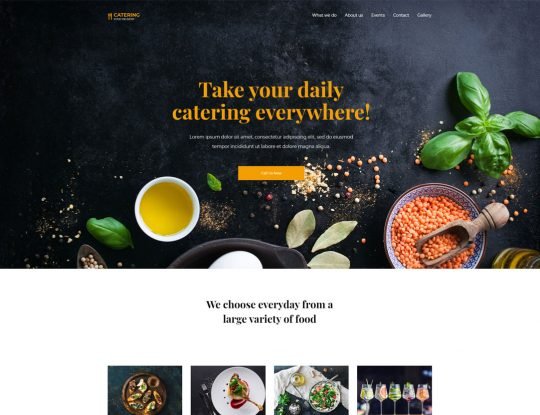The image appears to depict a website's landing page, likely focused on catering services. The backdrop is a stark black, which accentuates the vibrant colors of various elements and text scattered across the page. In the upper middle-left section of the screen, the word "Catering" is prominently displayed in a yellow-orange hue. Below this, there is a line of white text that is not entirely legible. Moving towards the center-right of the page, a navigation menu is visible, featuring the categories: "What We Do," "About Us," an unreadable option, "Contact," and likely "Delivery," all in white print.

Front and center, a powerful phrase commands attention: "Take Your Daily Catering Everywhere." The surrounding visual elements include a mix of spices, leafy greens (possibly spinach), an orange-colored pepper, and some pale green or nearly white leaves, adding a culinary touch to the page's aesthetic. The overall design suggests a visually appealing and comprehensive landing page tailored to a catering business.